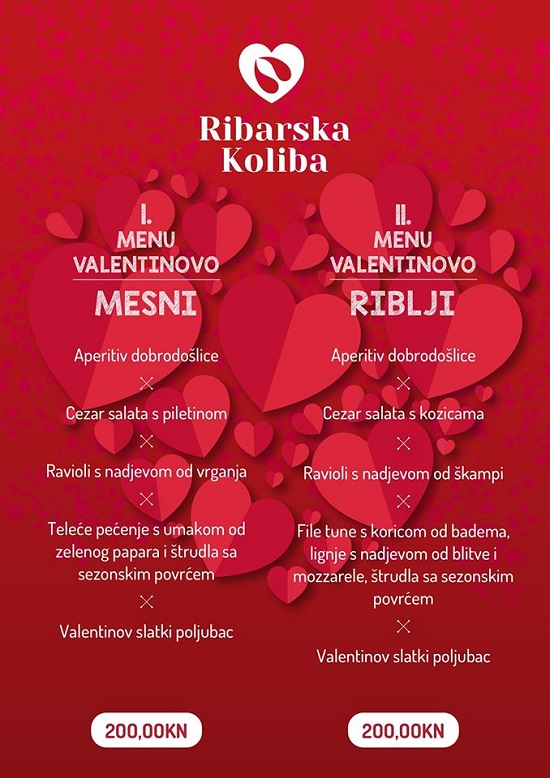The image portrays a Valentine's Day menu with a primarily red background, featuring a gradient from a brighter red at the top to a darker red at the bottom. Central to the design is a large heart formed by multiple smaller hearts, each displaying a two-tone color scheme of dark red on the left and lighter red on the right. Dominating the upper center of the image is a large white heart with two smaller red heart cutouts within it. Beneath this white heart is the text "Rybarska Koliba" written in a non-English language, suggesting the restaurant's name.

The menu is divided into two vertical sections. The left side is labeled "Menu Valentinova Mesni" and the right side is labeled "Menu Valentinova Riblji," indicating different menu options. Each section contains lines of text listing various items, and both sections culminate at the bottom with a white oval showing the price "200,000 Kn" in red text. This design, paired with the Valentine's Day theme, creates a romantic and festive presentation.